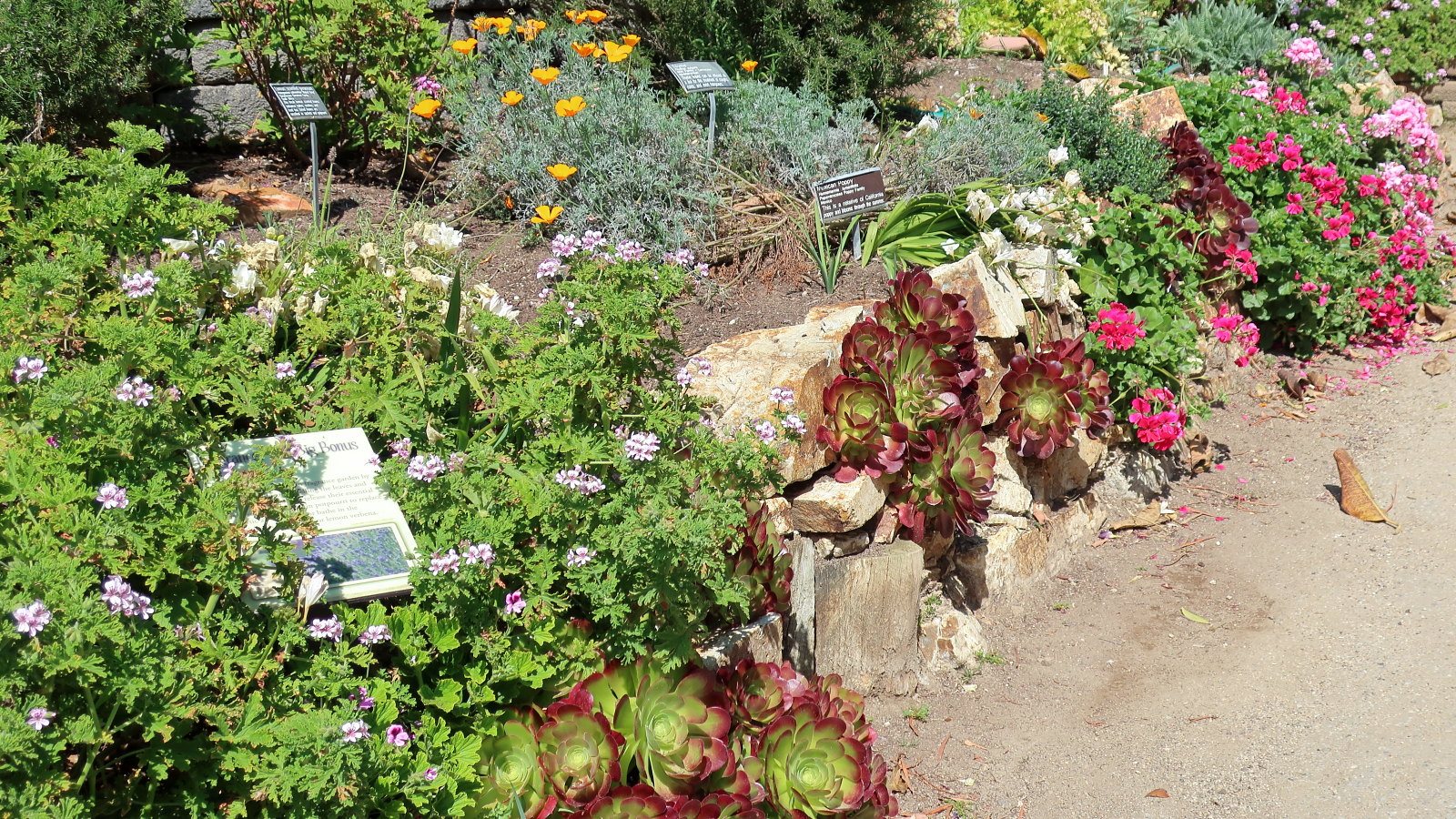This is an overhead photograph of a scenic rock garden, likely taken from an elevated viewpoint. The foreground features a dense green shrub adorned with light pink flowers on the left and a plaque with white and gray detailing nestled amongst the foliage. This plaque, intended to identify the plants, is positioned within an area of brown mulch. To the right of the shrub, you see a dirt pathway with a singular brown leaf lying on it.

Further into the mid-section of the image, a natural-looking ledge composed of white stones and large rocks is visible, creating a rustic, curved wall. Bright red and green flowers grow abundantly over this wall, adding vibrant contrast. Just behind this area, additional plaques with brown and gray backgrounds and white text provide further identification of the garden's botanical variety.

In the background, particularly to the upper left, another green shrub blooms with large yellow flowers, complementing the diverse floral tapestry of the garden. This area is bathed in sunlight, enhancing the lively colors of the foliage and flowers.

On the lower right corner of the photograph, an orange tabby cat sits on the brown dirt path, gazing curiously at the colorful display of flowers, contributing a charming touch to the serene garden scene.